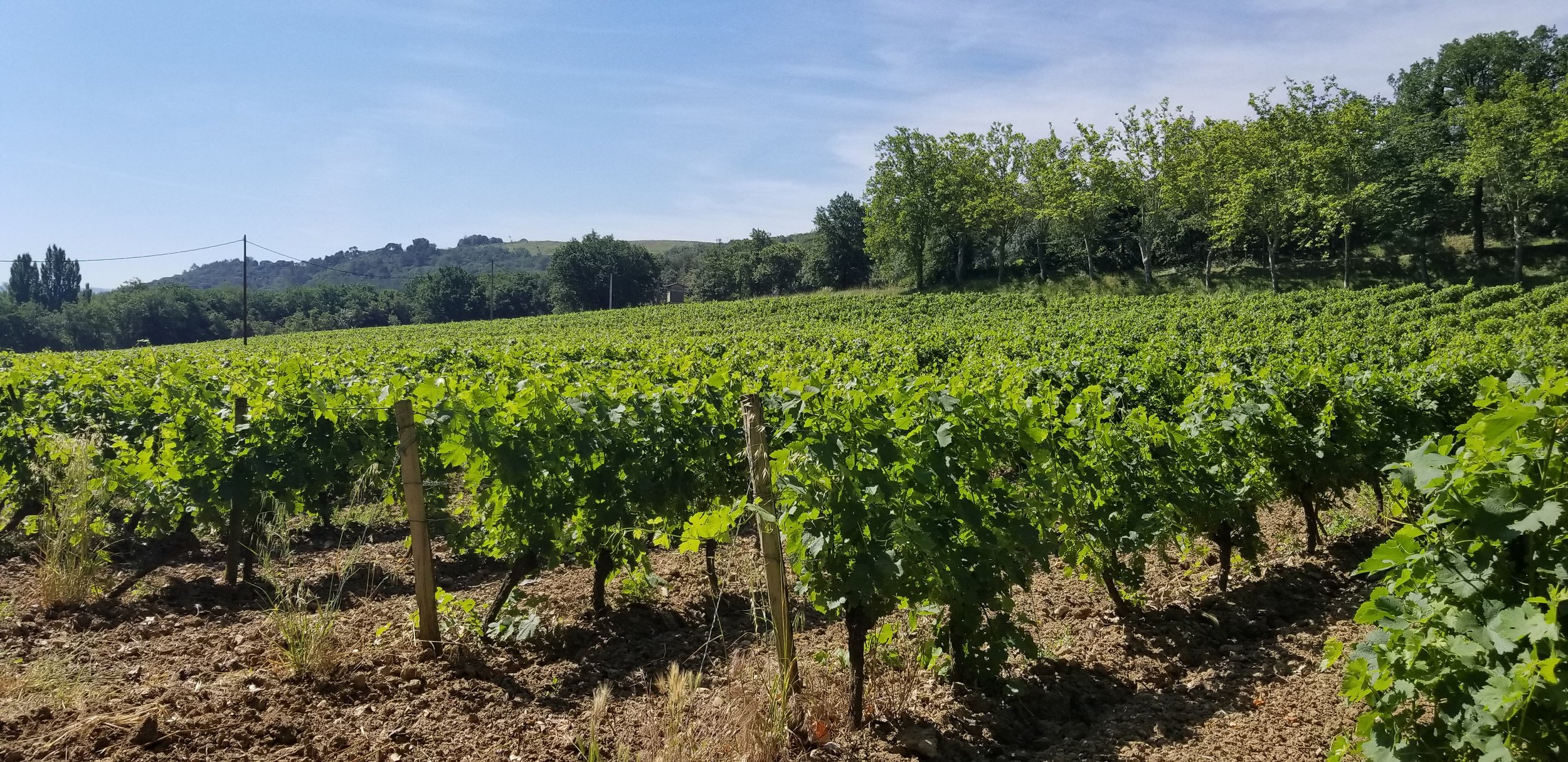In this photograph, taken outdoors during the daytime, we see an expansive vineyard stretching out before us. The image is rectangular, about six inches wide and two to three inches high. Captured from the end of the rows, we observe neat, orderly rows of bushy vineyard plants extending from the foreground to the distant background. Each row, planted in elevated mounds of dark brown soil, features a single light brown wooden stake marking its end and providing support to the nearest plant. The plants themselves, approximately two feet high, have dark green stalks with lush green grape leaves, which are irregularly shaped with sharp edges.

The field occupies the bottom half of the photograph, while the top half showcases a beautiful landscape. To the right are medium-sized, dark green deciduous trees, and to the left, a mountain or hillside area with power poles delineates the edge of the vineyard. The backdrop is a blue sky, accented by white clouds drifting from the right, lending a slightly hazy but distinctly sunny atmosphere to the scene. In the distance beyond the field, we can see rolling hills, adding depth and serenity to this vibrant agricultural setting.